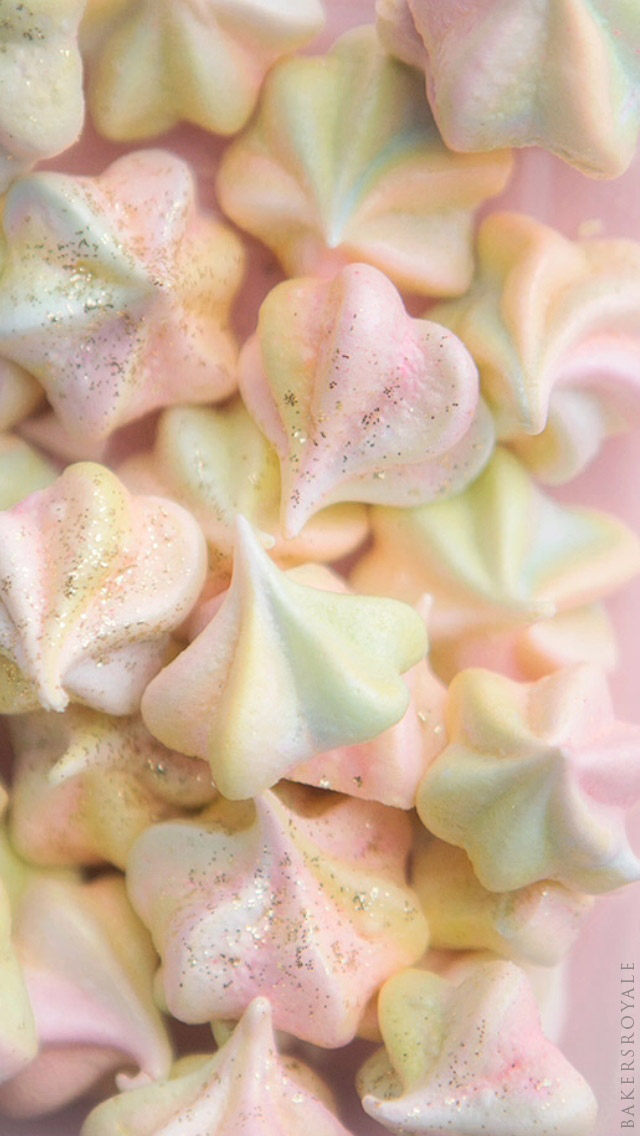This is a high-resolution, close-up, vertical portrait-oriented photograph of delicate meringue candies, piled in a random heap. The image focuses on their exquisite details, showing their piped star shapes with pointed tops. The candies appear in various pastel colors, predominantly pink, green, and light yellow, with occasional hints of blue and peach. Many of them are adorned with shimmering gold edible glitter, which sparkles under the light. The meringues are nestled against a light pink background, emphasizing their vibrant hues. In the bottom right corner, tiny grey text reads "BAKER'S ROYALE," written vertically up the side, signaling a possible advertisement or branded content. Overall, the image exudes an elegant and whimsical charm, suggesting these treats are a special, artisanal confectionery.